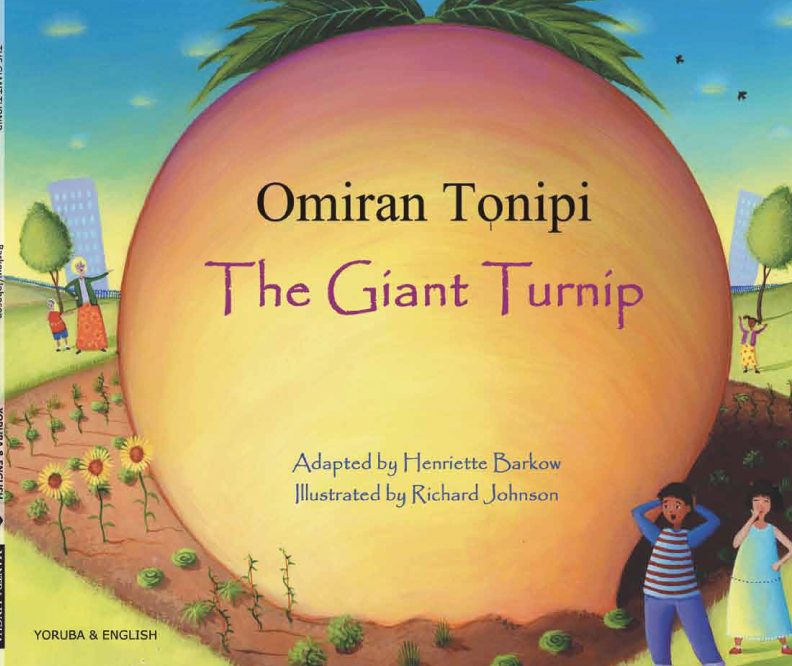The cover of the children's book "The Giant Turnip" by Omeran Tonipi features a colossal turnip dominating almost the entire garden patch, rendered in shades of rosy orange with purple shading around the edges and topped with vibrant green leaves. The garden area also includes sunflowers, leafy greens, and green beans on stakes. Surrounding the massive turnip are three children and an adult woman in a long flowery skirt. One little girl, wearing a purple sweater over a yellow and red dress, stretches out her arms in astonishment. A man in front, dressed in a red and white striped shirt, stands with his hands on his head, mouth agape in shock. In the background, additional figures can be seen amidst a tree and buildings, while a couple of black birds fly in the sky on the upper right. The title "The Giant Turnip" appears prominently on the turnip itself in large letters, with "Adapted by Henriette Barco" and "Illustrated by Richard Johnson" credited below. In the lower left corner, it also notes that the book is presented in both Yoruba and English.